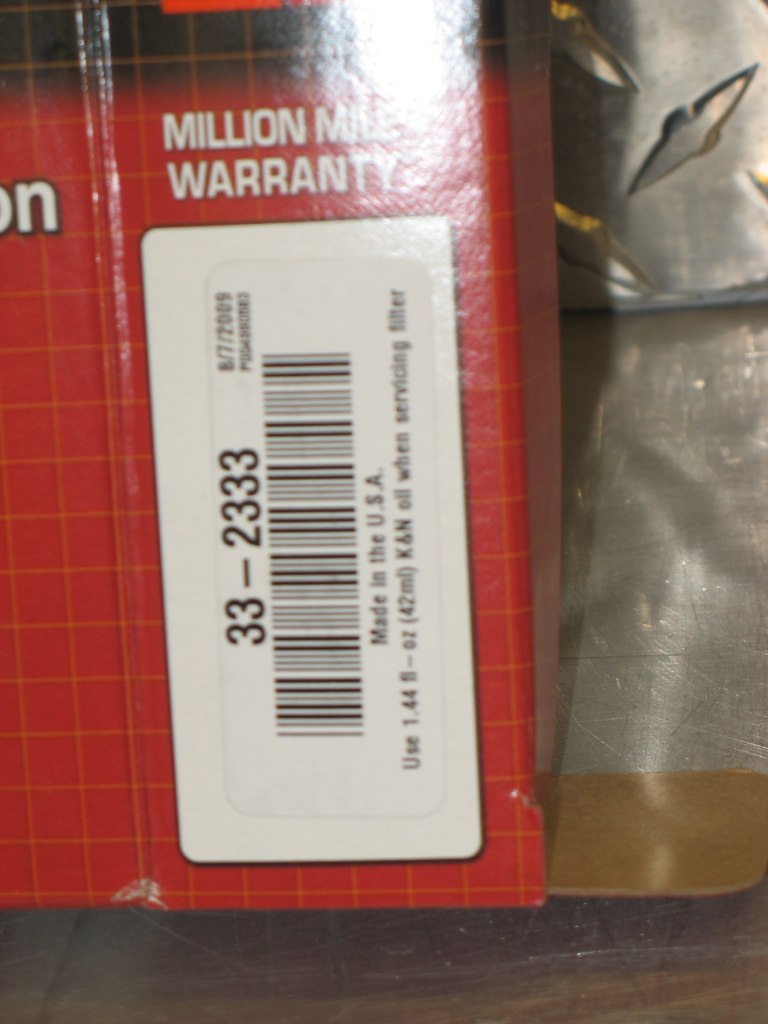The photograph depicts a barcode on a red and orange grid-patterned packaging, likely of an oil filter, resting on a metallic table, possibly in a workshop. The barcode is vertical and displays the numbers 33-2333. Above it, the text reads "Million Mile Warranty," and below it, there is additional information including "8th of the 7th 2009" and "Made in the USA." The surrounding environment includes some unspecified metallic pieces, enhancing the industrial atmosphere. The packaging includes some unreadable text, adding to the sense of mystery about the precise contents.